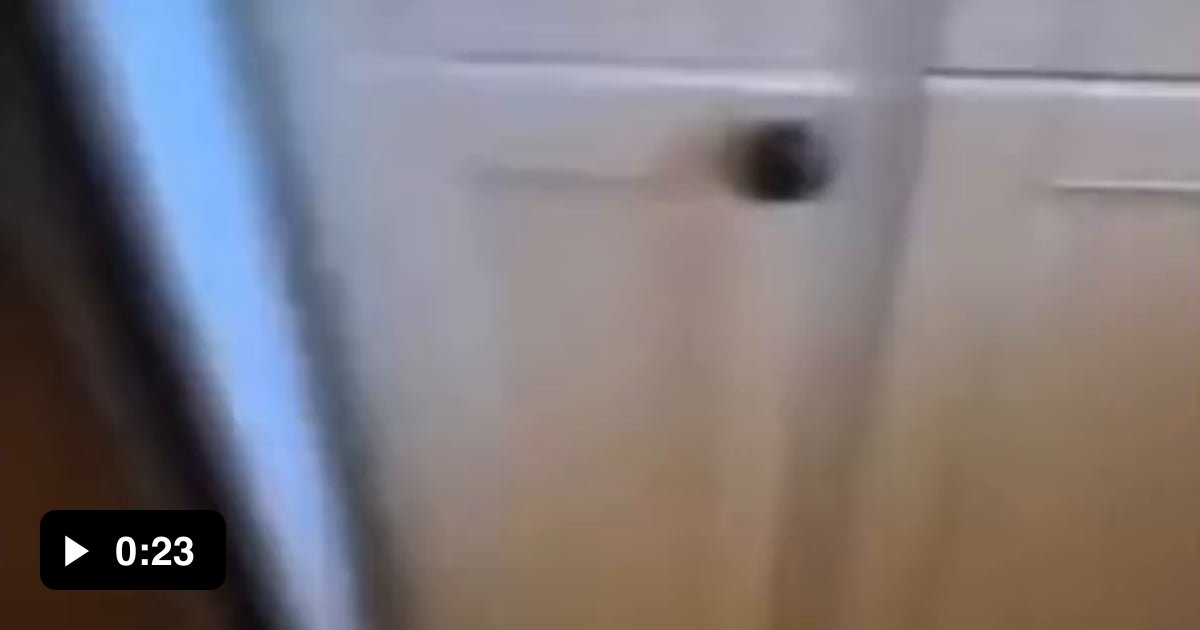In this image, the main focus is a slightly blurred close-up of a cabinet, which prominently features a dark brown handle. The door panels of the cabinet are light brown and rectangular, each with a detailed inset square. On the right side of the image, there's a black square overlay with white text indicating a timestamp of “0.23 seconds.” The left side of the image fades into a bluish-white hue, potentially hinting at another black-colored door just off to the side. The overall lighting and slight blur suggest a hurried or candid capture, adding an element of spontaneity to the scene.